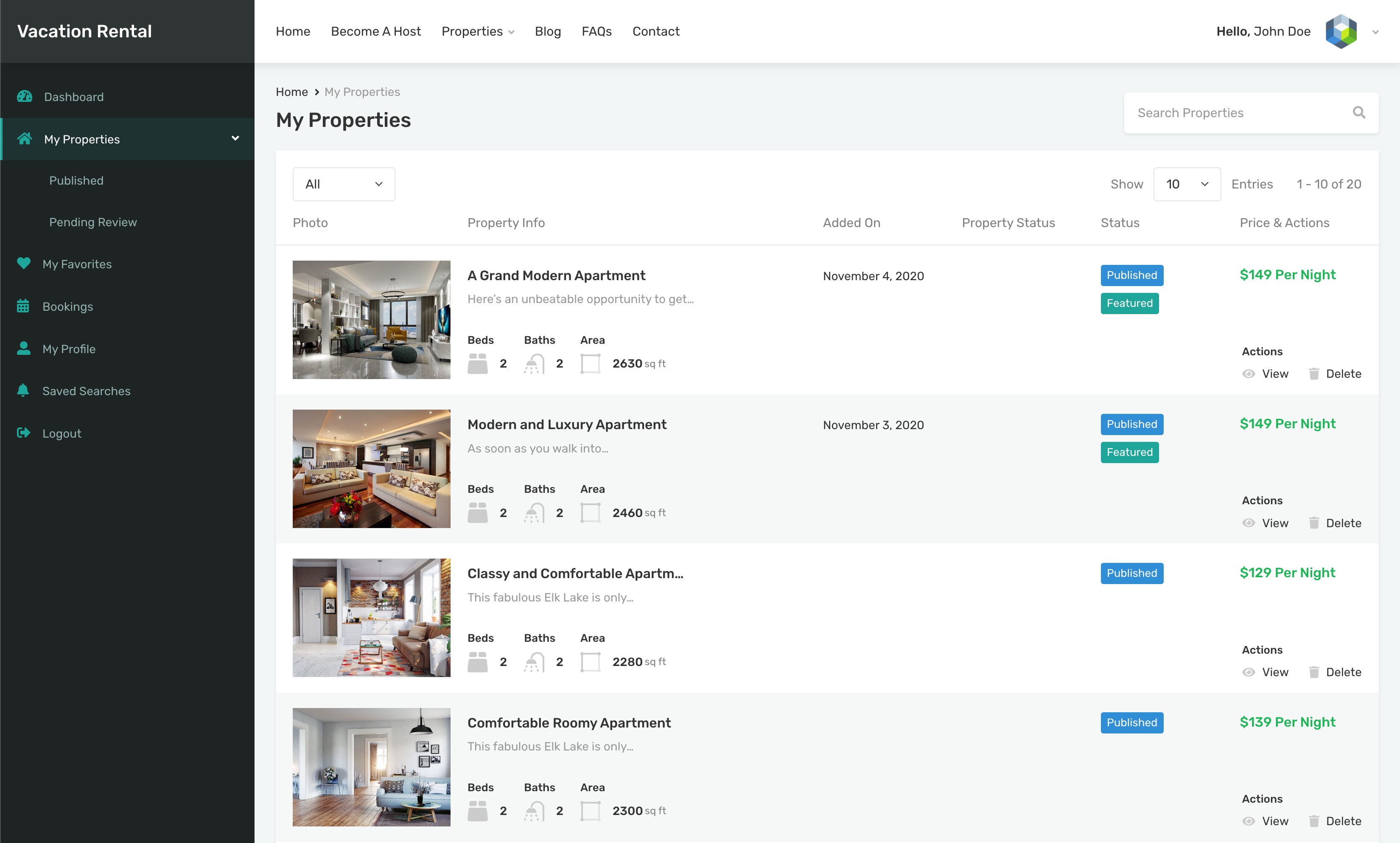The image displays a website interface for managing vacation rental properties. On the left side, there's a vertical black menu banner that transitions from a lighter shade of black at the top to a darker shade at the bottom. At the top of this banner, "Vacation Rental" is written in white print. Below, there are turquoise icons aligned to the left, followed by white text labels for different menu items including "Dashboard," "My Properties" (which has a drop-down menu revealing "Published" and "Pending Review"), "My Favorites," "Bookings," "My Profile," "Saved Searches," and "Logout."

On the main section of the website against a white background, a horizontal navigation bar is present at the top displaying "Home," "Become Host," "Properties" (with a down arrow indicating a drop-down menu), "Blog," "FAQs," and "Contact."

Further to the right side of the interface, the user is greeted with "Hello, John Doe" against a light gray background. Below this greeting, navigation breadcrumbs are shown: "Home" followed by a right arrow leading to "My Properties." Under these breadcrumbs, the main heading "My Properties" is displayed in larger black text.

To the right, a search bar with a "Search Properties" placeholder and a magnifying glass icon allows users to search properties. Below the search bar, there's a filter section with "All" in a drop-down menu, followed by sorting options labeled "Photos," "Property Info," "Added On," "Property Status," "Status," "Price," and "Actions." A control labeled "Show 10" with a drop-down menu option indicates the number of entries displayed per page, and a note shows "Entries 1-10 of 20."

Within the property listing area, four properties are displayed: "A Grand Modern Apartment," "Modern and Luxury Apartment," "Classy and Comfortable Apartment," and "Comfortable Roomy Apartment."